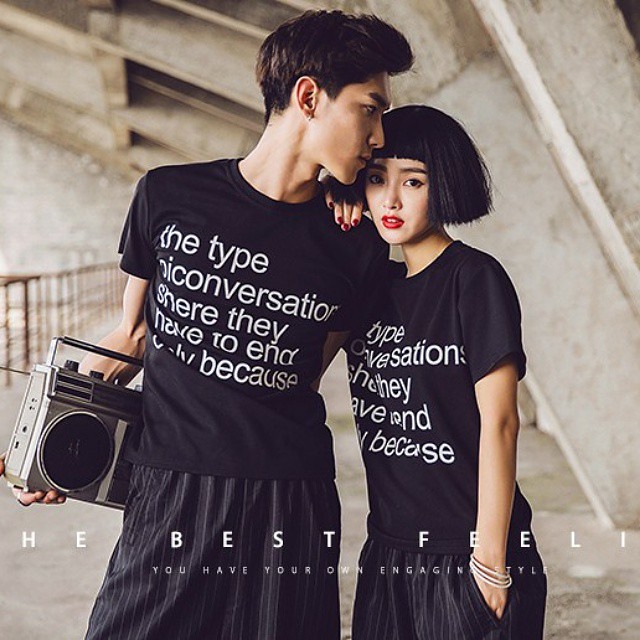This photograph appears to be an outdoor fashion advertisement featuring two young Asian models in their early twenties, dressed in matching outfits. They stand against a concrete background with a vaulted ceiling and a railing on the left, creating a grayish, industrial ambiance. Both models wear identical black short-sleeved t-shirts with white lettering that reads, "The type of conversation they share have to end only because," though the text is partly obscured by folds in their shirts. The t-shirts are paired with loose, black pants adorned with gray pinstripes. 

The male model, positioned on the left, holds a large, old-fashioned silver boombox with a cassette player, resting it on his hip while looking to the right. He has medium-length brown hair. The female model, on the right, has a sleek black bob hairstyle and is leaning against the man, one hand resting on his shoulder and the other in her pocket. She is also wearing bangles on her wrist. At the bottom of the image, there is an additional caption in white text that reads, "The best feeling, you have your own engaging style." The overall scene suggests a retro and stylish vibe, emphasizing the connection and shared fashion sense between the two models.